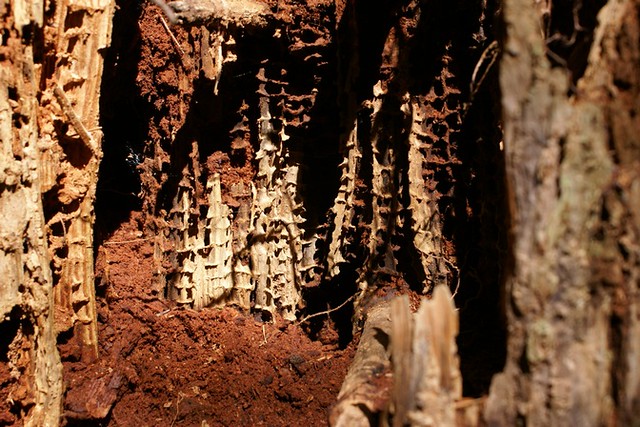The image appears to be an intriguing natural scene that could either be a dense, earthy woodland area or the interior of a cave. Dominated by rich, brown and clay tones, the scene features a middle section where fragmented tree trunks or potential stalagmite-like formations are prominently displayed. These formations, white and brown in color, might be shreds of trees that have either deteriorated or been uniquely carved by nature, giving them a statue-like appearance. Surrounding these central growths, the ground is covered in brown mulch and soil. The left side of the image reveals what seems to be an opening within a tree trunk, while the right side shows blurred textures that resemble tree bark. Shadows cast over the area add a layer of depth, enhancing the mysterious and earthy ambiance of the scene. The details hint at a complex interaction between natural decay or sculpting, with elements that may be earthy stalagmites or simply tree growths, contributing to the overall enigmatic beauty.